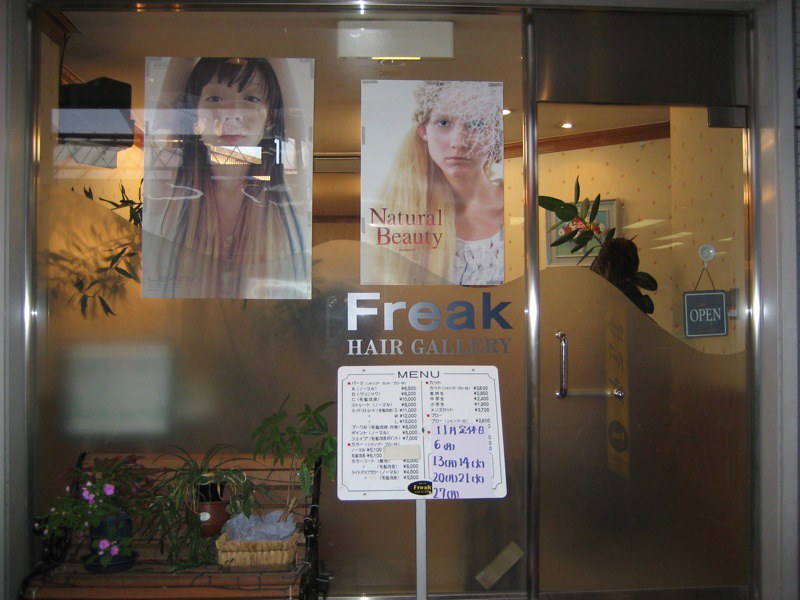The image shows the exterior of a beauty salon named "Freak Hair Gallery," with the name displayed in a gradient of dark blue to light silver text. The storefront features a large glass window divided into two sections: the lower half has frosted glass creating a wave pattern, and the upper half is clear. To the right of the window, there is a door sharing the same glass design. Below the "Freak Hair Gallery" sign, a smaller square sign labeled "Menu" lists the salon's services and prices in what appears to be Japanese text, though it is hard to read.

Displayed prominently on the glass window are two posters. The left poster features an Asian woman with black hair styled with faded streaks of red and yellow, wearing a horizontally striped dress in blue, red, and yellow hues. Her arms are raised, showcasing her armpits, but there is significant glare from the glass which partially obscures the image. The right poster depicts a blonde woman with long hair labeled "Natural Beauty" in red text. She is dressed in a white shirt and looks directly at the camera.

Adjacent to the window rests a bench made from horizontal wooden planks, with black metal armrests. On the bench are several potted plants, with pots ranging in color from brown to dark blue, as well as a small basket. The environment also includes an "Open" sign in dark blue with white text located near the door, indicating the salon is operational. The entire setting has an inviting yet mysterious ambiance, blending various colors and textures.